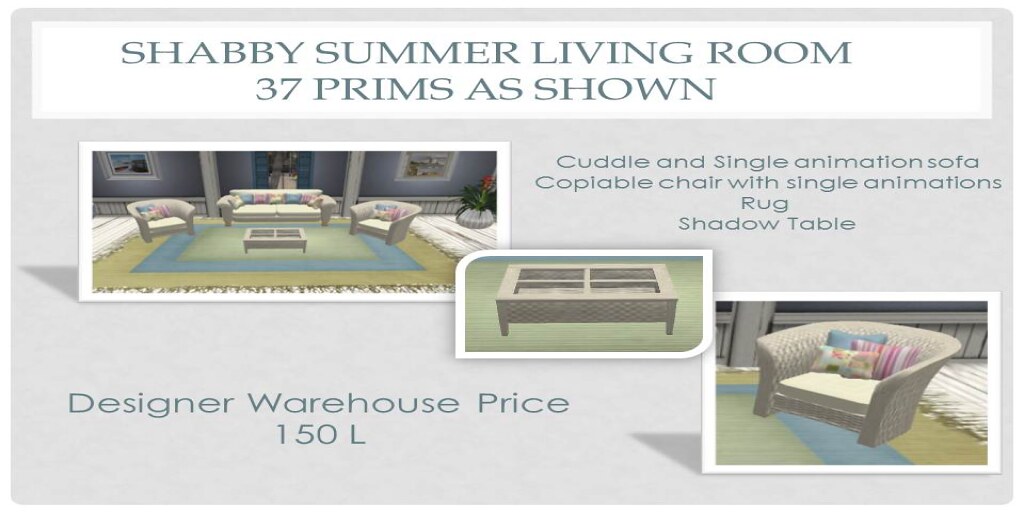This rectangular advertisement promotes a "Shabby Summer Living Room" furniture set for a video game. The top features a white banner with blue text reading "Shabby Summer Living Room, 37 Prims as shown." Below this, the image showcases three digital photographs arranged diagonally from the top left to the bottom right.

The largest photo on the left illustrates a cozy living room setting. It includes a 3D rendered double-seated couch flanked by two identical armchairs, all placed on a tan and blue rug. A white coffee table with a glass, window-style surface sits in the center. Additional decor items like wall art and a potted plant accentuate the pastel-colored, light and airy room.

To the right of this main photo, smaller images provide close-ups: one highlights the detailed design of the coffee table, with its textured sides and glass panes, while the other zooms in on an armchair, revealing its club shape, bottom cushion, and four decorative pillows.

Adjacent to these images, a blue font description lists the items: "Cuddle and Single Animation Sofa, Coppola Bowl Chair with Single Animations, Rug, Shadow Table." The text aligns with the cohesive aesthetic of the set.

At the bottom, another blue font note reads "Designer Warehouse Price 150 L," implying the cost. The overall background of the advertisement is a light blue shade, enhancing the summery vibe of the furniture set.